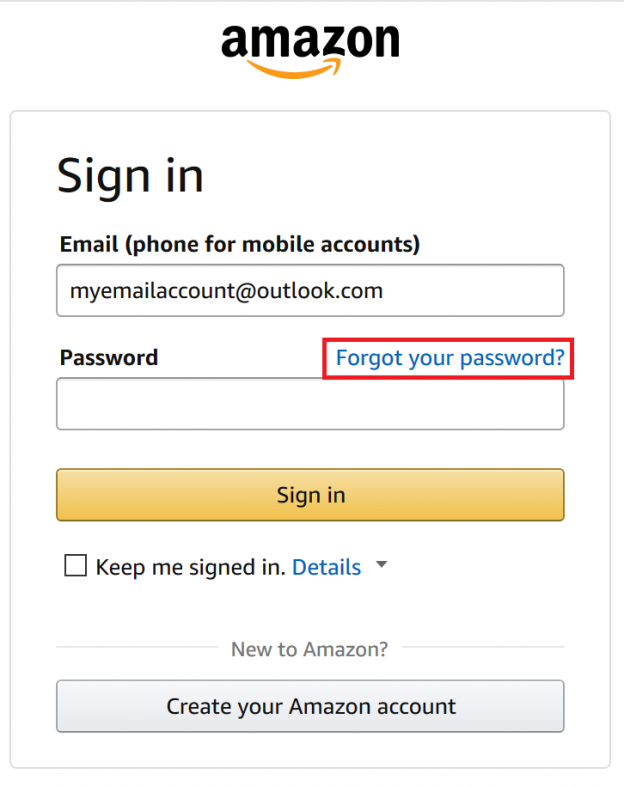Here is the cleaned-up and detailed caption for the image:

---

The image depicts a typical Amazon sign-in page. At the very top, the word "AMAZON" is prominently displayed in a black, capitalized font. Below this, the distinctive Amazon swoosh is rendered in gold, completing the recognizable Amazon logo. 

This logo and text are enclosed within a thin, square border. Inside this border, the first item is the header "Sign-In," with the 'S' capitalized. Below this, there is a double space followed by the label "Email (phone for mobile accounts)" in dark black font. 

A rectangular text box follows, containing the email address "myemailaccount@outlook.com" and bordered in gray. Below this email field, the word "Password" appears in a dark print. On the same line, towards the right, a blue, clickable "Forgot your password?" link is outlined by a red-bordered box.

Beneath this link, there is a larger box for entering the password. Following this, there is a gold-colored rectangle with the text "Sign-In," where the 'S' is capitalized, written in black font. 

Below this, there is a checkbox option labeled "Keep me signed in," accompanied by a clickable link titled "Details." 

Lastly, at the bottom of the page, in a lighter gray font, the phrase "New to Amazon?" is posed as a question. Next to it, a clickable, rectangular box reads "Create your Amazon account."

---